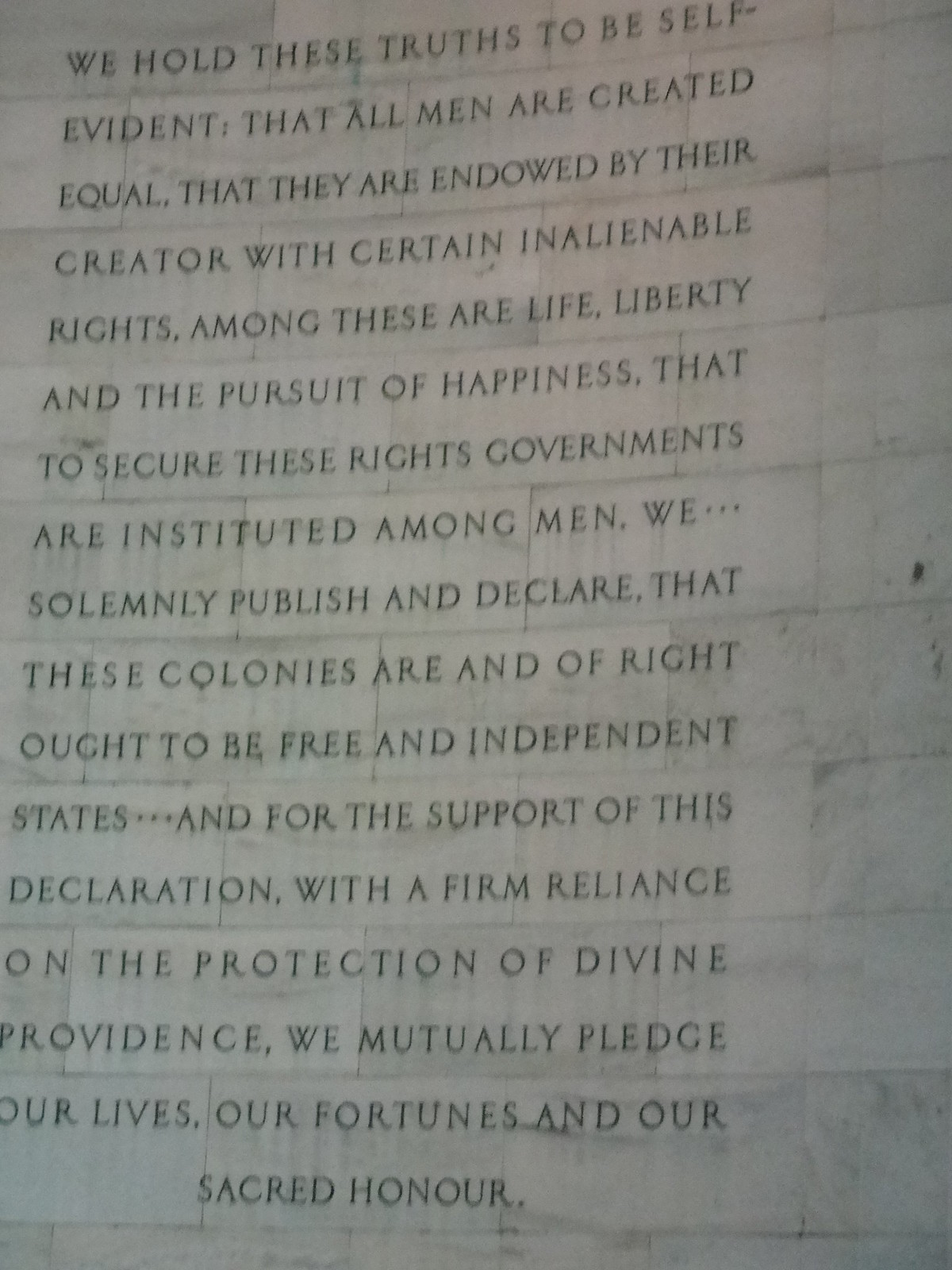The image depicts a marble monument, likely situated in Washington, DC, featuring an extensively inscribed wall. The backdrop appears light green, segmenting the text into sections, but the engraving spans the entire visible surface. The text, carved in black, all-capital serif font, declares foundational principles of American independence. It begins with "We hold these truths to be self-evident, that all men are created equal, that they are endowed by the Creator with certain inalienable rights. Among these are Life, Liberty, and the pursuit of Happiness. That to secure these rights, governments are instituted among men." It continues with, "We solemnly publish and declare that these colonies are, and of right ought to be, free and independent states. For the support of this declaration, with a firm reliance on the protection of divine providence, we mutually pledge our Lives, our Fortunes, and our sacred Honor." The text's rectangular arrangement flows across the monument, emphasizing the gravity and enduring significance of the inscribed declaration.